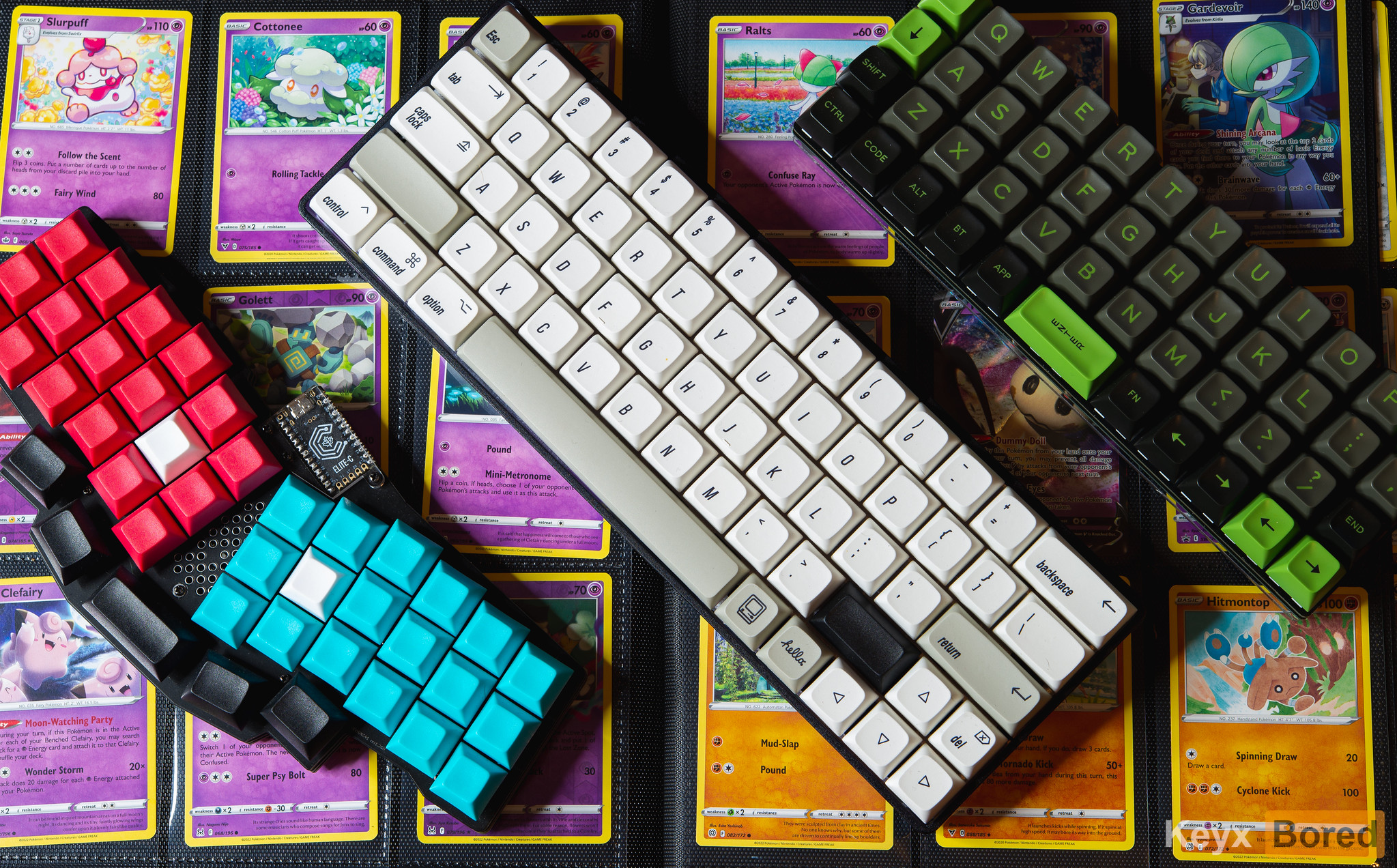In this image, three keyboards are diagonally arranged from the upper left to the bottom right against a background of Pokémon-style trading cards. Starting from the bottom left, there is a wavy ergonomic keyboard featuring red keys on the left and blue keys on the right, all tilted at an angle, enclosed in a black frame. In the middle, a traditional white QWERTY keyboard with black trim features a mix of white and gray keys, where specific keys like delete, backspace, spacebar, and shift are gray. In the upper right, the third keyboard, presumably from Razer, has a black base with highlighted lime green keys, including directional arrow keys, and gray keys bearing lime green lettering. The background consists of an open file holding nine trading cards on each side, for a total of 18 cards. The cards on the left half primarily display a purple background, while the cards on the right half are split between purple and orange backdrops. Each card prominently features an image and various attributes such as levels of skill, resembling the detail and style of traditional Pokémon collectible cards.